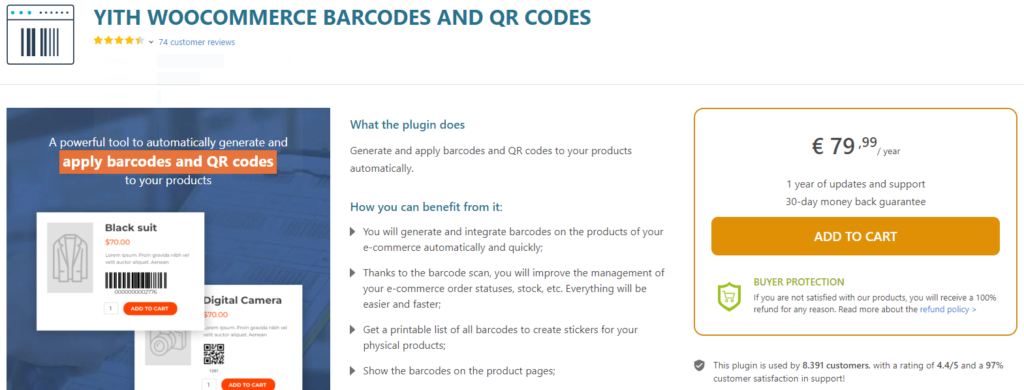Image Description:

The image showcases a product page against a white backdrop. 

**Top Left Section:**
- A small black box in the upper left-hand corner features three green circles on the left and six black circles on the right, separated by a thin black line. Below the line, there is a barcode-like series of lines: three black on the left, a small white gap, two black, and three gray lines flush right.

**Header Text:**
- To the right, in blue text, it reads: "YITH WooCommerce Barcode and QR codes." Below this, a five-star rating is depicted with three and a half stars lit up. Adjacent to this is a drop-down arrow, and in blue text, it says "74 customer reviews."

**Main Content Area:**
- Below the header, a small gray line runs across the width of the page.
- In the left-hand corner, a blue box contains white text: "A powerful tool to automatically generate." Beneath this, in a green box with white text, it says, "Apply barcodes and QR codes," followed by white text stating, "to your products."

**Product Cards:**
- Two white product cards are displayed, the left one overlapping the right one slightly. Each card has a small black and gray box in the upper-left corner.
  - The top card shows an outline of a gray coat with the text "Black Suit" above it in black. Below that, "$20" is displayed in orange, followed by two lines of black text and a barcode image. A red bar on the right states "Add to cart" in white.
  - The bottom card features an outline of a black camera. "Digital Camera" is written in black at the top, with "$70" in orange underneath. Two lines of black text and a QR code follow. An orange bar on the right reads "Add to cart" in white.

**Center of the Page:**
- Blue text at the top center explains the plugin's purpose: "Generate and apply barcodes and QR codes to your products automatically."
- Below this, a headline in blue reads, "How you can benefit from it."
- Four bullet points, each marked by a small black right-pointing arrow rather than a circle, are listed:
  1. "You will generate and integrate barcodes on the products of your e-commerce automatically and quickly."
  2. "Thanks to the barcode scan, you will improve the management of your e-commerce order statuses, stocks, etc. Everything will be easier and faster."
  3. "Get a printable list of all barcodes to create stickers for your physical products."
  4. "Show the barcodes on the product page."

**Right Sidebar:**
- A white box highlighted with a thin yellow line features a price, marked by a pound symbol followed by "79.99/year." Beneath, centralized black text states: "One year of updates and support," followed by, "30-day money-back guarantee."
- An orange bar below this reads "Add to cart" in white.
- Further down, a shield outlined in green contains a green card icon. Next to it, in black text, it reads "Buyer Protection," followed by more text explaining: "If you are not satisfied with our product, you will receive a 100% refund for any reason." The phrase "refund policy" at the end is in blue, denoting a clickable link.